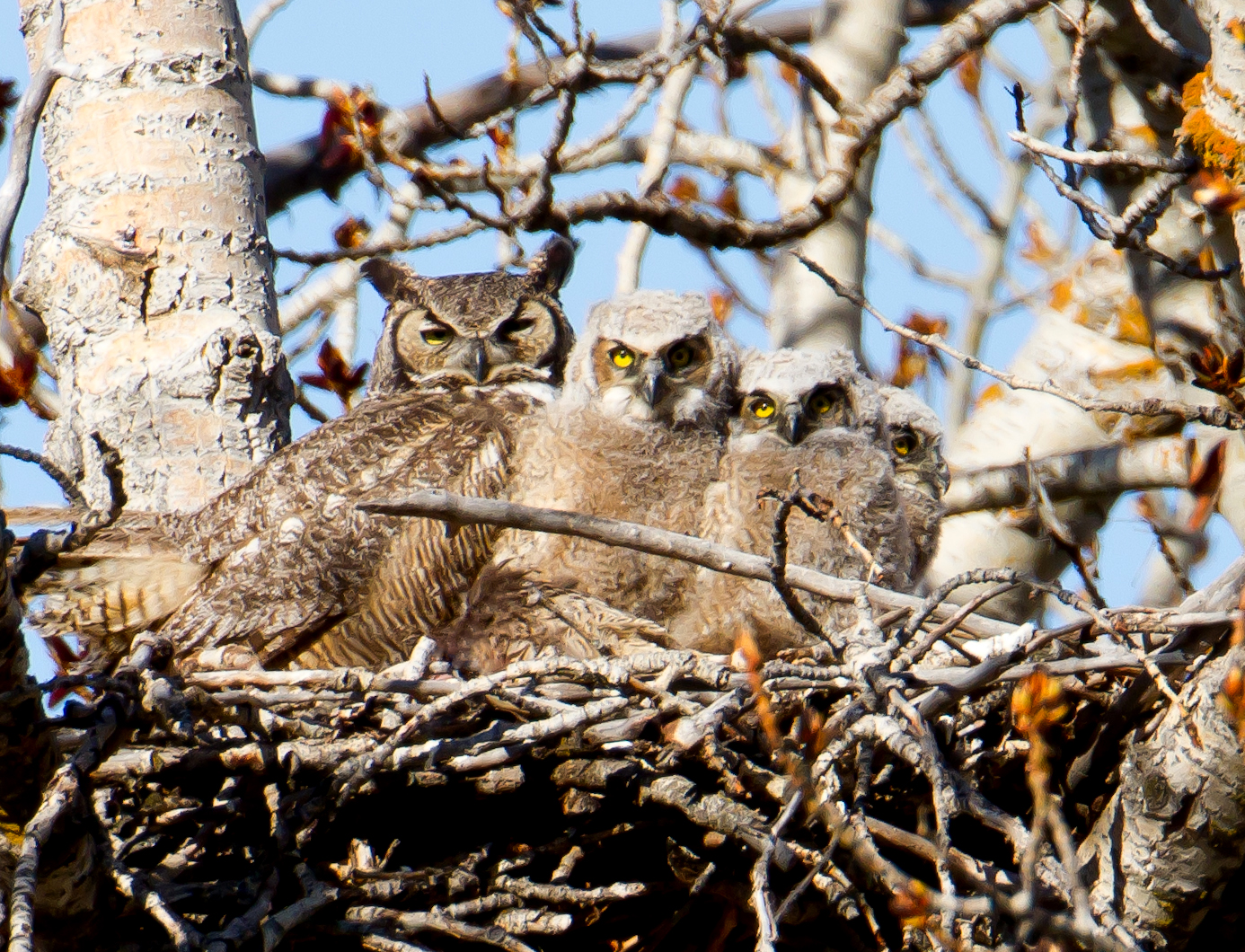The image is a professional, rectangular, horizontally-oriented photograph capturing a family of owls nestled in a tree nest against a clear, light blue sky. The scene is set during the daytime and the nest is composed of various brown and gray sticks and twigs, supported by light brown tree branches largely devoid of leaves, suggesting a winter setting. 

Front and center are four owls. The adult owl on the left, notable for its darker brown feathers and a bit of white around the head, has partially closed eyes, but the yellow can still be seen. The adult owl also has longer feathers. The three smaller owls, likely its offspring, have white heads and lighter brown bodies, with conspicuous yellow eyes. Each owl is positioned distinctively – three of them face the camera directly, while the fourth owl looks to the right. The color palette of the scene encompasses shades of yellow, brown, gray, black, and hints of orange, enhancing the natural and serene atmosphere of the photograph.